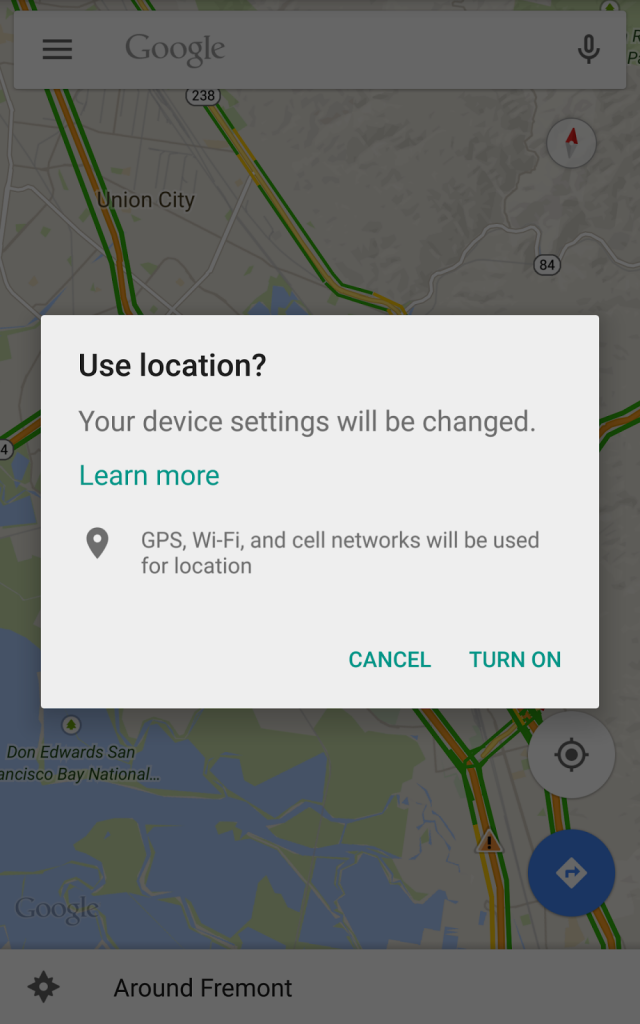A screenshot of a mobile phone displaying the Google Maps application. In the foreground, there is a prominent pop-up message from Google asking for location permissions. The message states, "This device would like to use your location," and provides an explanation about the services needing location access for better functionality. It offers two choices at the bottom: "Cancel" or "Turn On."

The pop-up appears in the middle of the screen, slightly obscuring the underlying map. At the top of the screen, the Google logo is visible, indicating the active application. Beneath the pop-up, the map shows a section of Union City, including major freeways and a nearby water body. At the bottom of the screen, text reads "Around Freeman," suggesting the current area of interest or search. The screenshot highlights the necessity of enabling location services for improved navigation and assistance features in the Google Maps app.